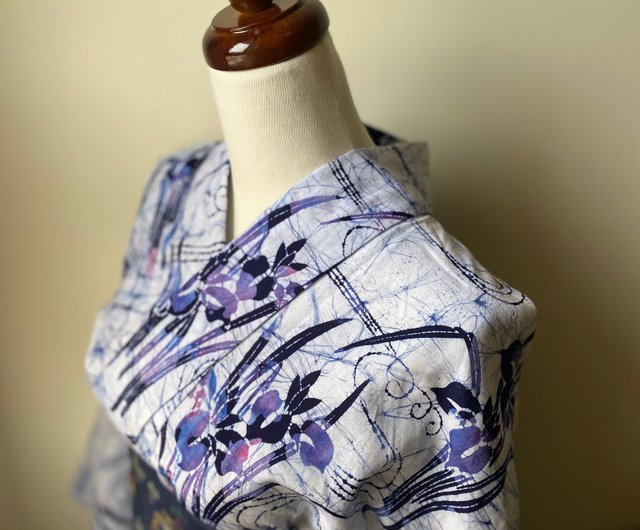This detailed photorealistic picture, taken indoors, captures a headless, highly polished dressmaker's mannequin with a glossy, brushed dark wooden joint at the neck. The mannequin, with its cream-colored tone, is adorned with a garment that ambiguously resembles a kimono, shirt, or dress, characterized by a wide collar and potentially three-quarter or full-length sleeves. The garment draped over the mannequin displays a delicate pattern featuring blue and purple flowers along with dark blue leaves or stems on a light-colored background, specifically white or light blue to cream or light tan. The light source, coming from the left, casts the mannequin's shadow to the right, highlighting the intricate stylized floral design that does not repeat, creating a unique and expensive look to the ensemble.